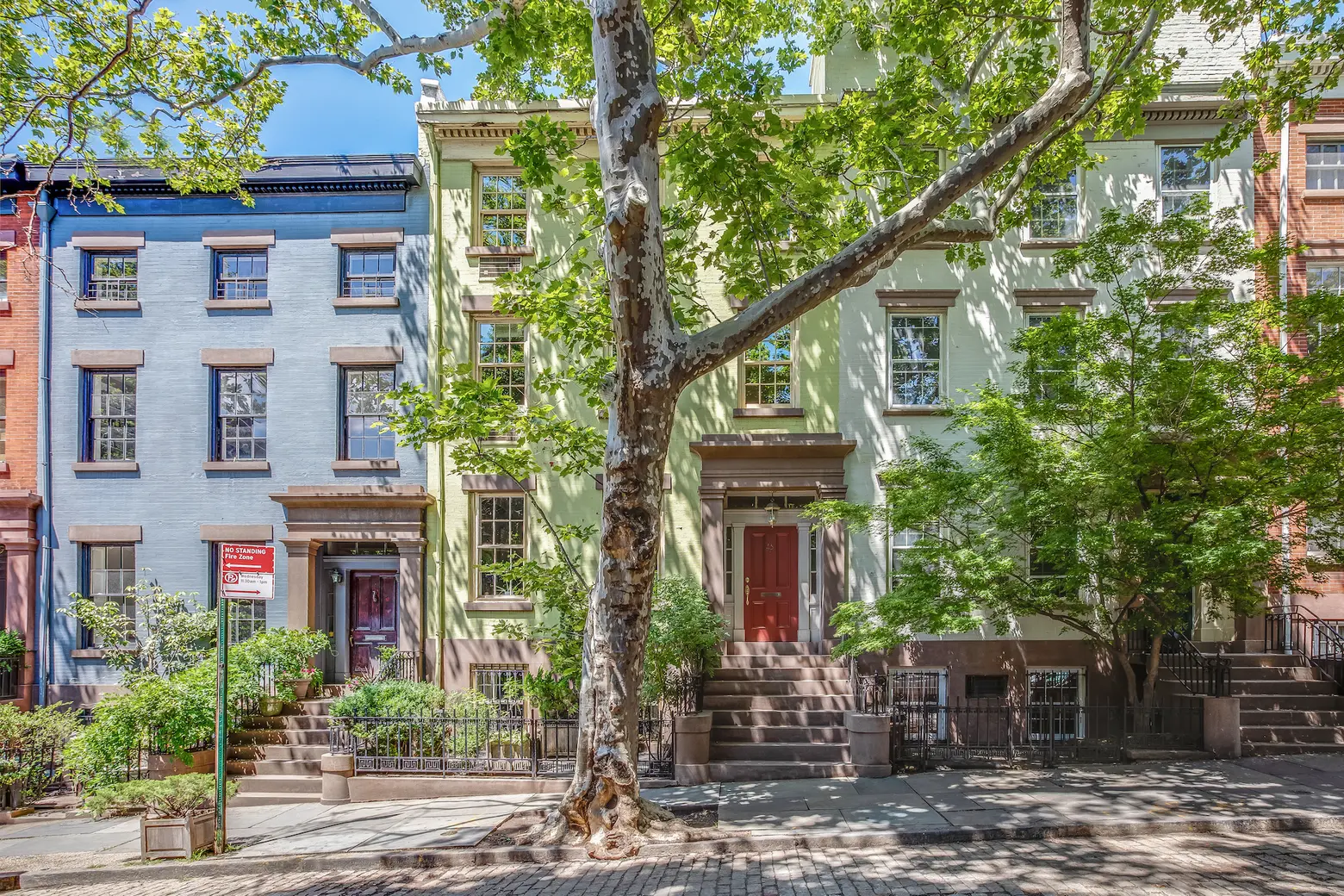The image depicts a photorealistic, city apartment scene with a straight-on view of several attached, three-story buildings flanked by large trees casting shadows on the sidewalk. From left to right, there is a partially visible pinkish apartment, followed by a blue one with windows framed in gray trim. Next is a beige or cream-colored building in the center, featuring a prominent tree with visible roots breaking through the sidewalk. This tree has a creamy appearance with brown spots and lush green leaves. Further to the right, there is a white apartment with a smaller tree in front, followed by a peach-colored building that extends off to the side. All buildings appear to have concrete stairs leading up to variously colored front doors—red, brown, and yellow—with cast iron railings in between. A green metal street sign post near the trees holds a red and white sign that reads "No Standing Fire Zone." The sky above is clear and blue, enhancing the vibrant colors of the buildings.